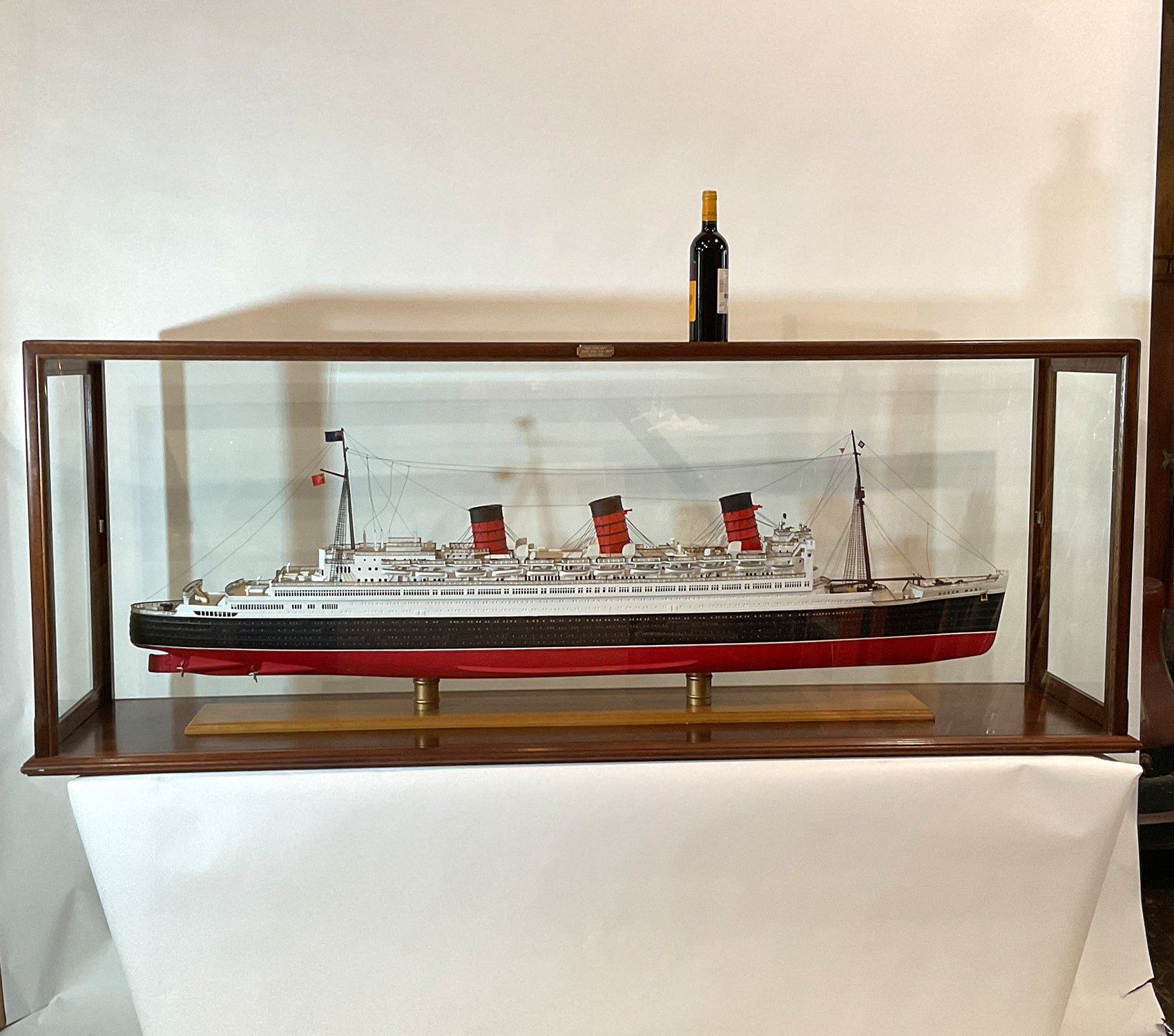The photograph showcases a large glass display case made of dark oak wood with polished edges. The display case has glass panels on all sides and possibly a small brass plaque on the top. Inside, there is a meticulously built model ship that resembles the Titanic. The model ship has a white upper deck, a black midsection, and a red keel that would be submerged underwater. There are three prominent smokestacks (steam stacks) with red bottoms and black tops. The ship features detailed rigging lines extending from masts at the bow and stern, as well as numerous tiny lifeboats and windows, adding to the intricacy of the model. The ship is elevated on two bronze-colored, spool-shaped supports and set on a slightly lighter oak wooden base within the display case. The entire case appears to be placed on a raised platform or table draped in what looks like white paper or a tablecloth. Atop the display case sits an unopened bottle of wine with a yellow and white label and a yellow foil around its neck. The display case, bottle of wine, and their shadows create a cohesive, yet complex visual against a background that matches the draped surface beneath the case.